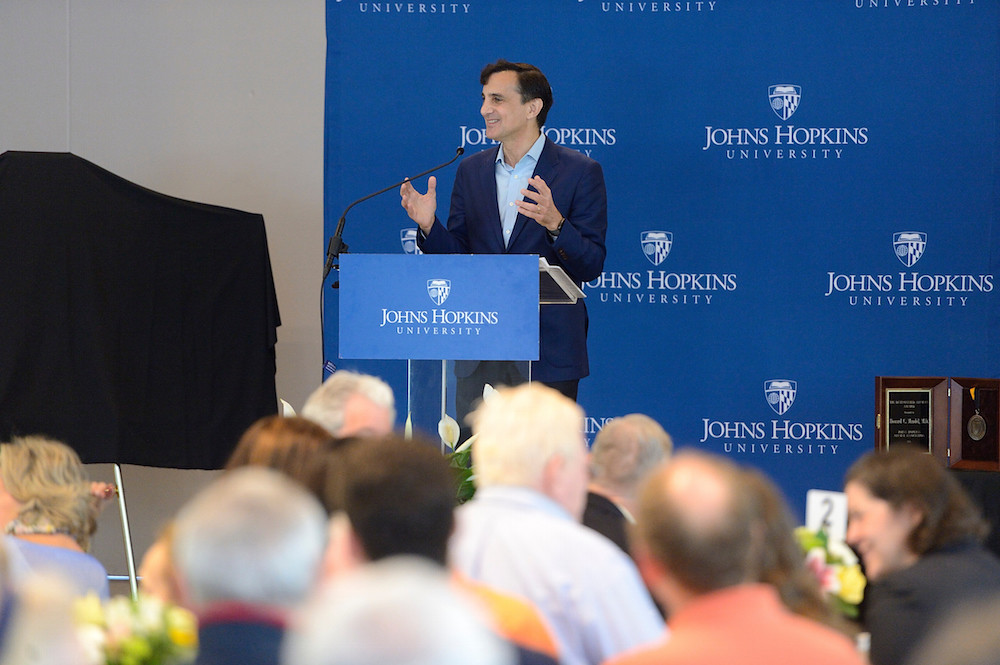In this detailed photograph taken during a live event at Johns Hopkins University, a man with short brown hair is prominently featured at the center, standing behind a podium. He is wearing a light blue collared shirt paired with a dark blue suit jacket, and black pants, speaking into a black microphone attached to the podium. The podium itself displays a blue sign with the Johns Hopkins University logo, complete with an emblem above it and smaller text underneath.

The backdrop behind him is a repetitive dark blue board adorned with the Johns Hopkins University logo and insignias in white. This creates a consistent branded background. To the left of the man, there is an easel draped with a black cloth, adding an element of intrigue. The setting includes a gray wall behind him to the left.

In front of the man, a large crowd is seated, their figures slightly blurred to emphasize the speaker. The audience mostly shows the backs of their heads, but a woman with brown hair in the bottom right corner is visible in profile, glancing to the left. Just above her, a plaque is noticeable on a table, situated on the stage in the background.

This image effectively captures the essence of a formal speaking engagement at Johns Hopkins University, with a focus on the man addressing the attentive audience.